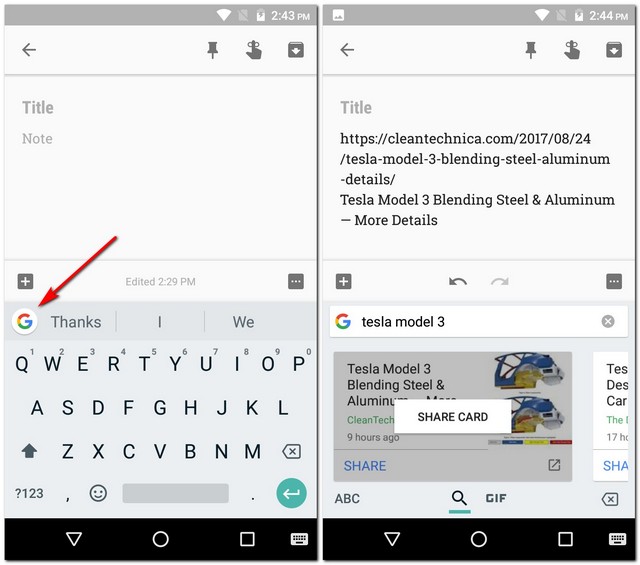Here are the cleaned-up and detailed descriptions of the two screenshots side-by-side on a mobile device:

---

**Left Screenshot:**

The timestamp on the screenshot reads "2:43 PM", displayed in the grey bar at the top, which also contains icons for WiFi, battery charge, and other status indicators. Below this bar, a left-facing arrow and a pushpin icon are aligned to the right, all in dark grey. There is also a forefinger with a ribbon icon, symbolizing a reminder, followed by a file icon with a downward arrow indicating a download option. 

Beneath this row of icons is a thin line, under which the screen displays fields labeled "Title" and "Note". These fields are empty, occupying the upper half of the screen. The lower half of the screen features the QWERTY keyboard, with a large red arrow pointing to the multicolored "Google G" icon located at the top left of the keyboard. The keyboard also includes the buttons "Thanks", "I", and "We".

At the bottom of the screen, the standard black navigation buttons for the smartphone are visible. An overlay notes that the screen was edited at "2:29 PM".

---

**Right Screenshot:**

The timestamp on this screenshot reads "2:44 PM", visible in the same grey bar at the top with similar status icons for WiFi, battery charge, and more. Similar to the left screenshot, a left-facing arrow and a pushpin icon are aligned to the right below this bar, followed by a reminder icon and a download icon.

This screen features a field labeled "Title", which contains the text "cleantechnica.com". Below this title is a secure URL for a website related to Tesla Model 3. The lower portion of the screen displays an active Google search result listing for "Tesla Model 3", with the description mentioning the blending of steel and aluminum, posted by Cleantech nine hours ago. A white box labeled "Share Card" is superimposed on this search result.

It appears that the user clicked on the "Google G" icon from the keyboard on the left screen, leading to Google search results displayed on the right screen. At the bottom of this screenshot, the standard black navigation buttons for the smartphone are also visible.

---

These detailed captions describe not only the elements present in the screenshots but also the sequence of actions taken by the user, providing comprehensive context for the images.